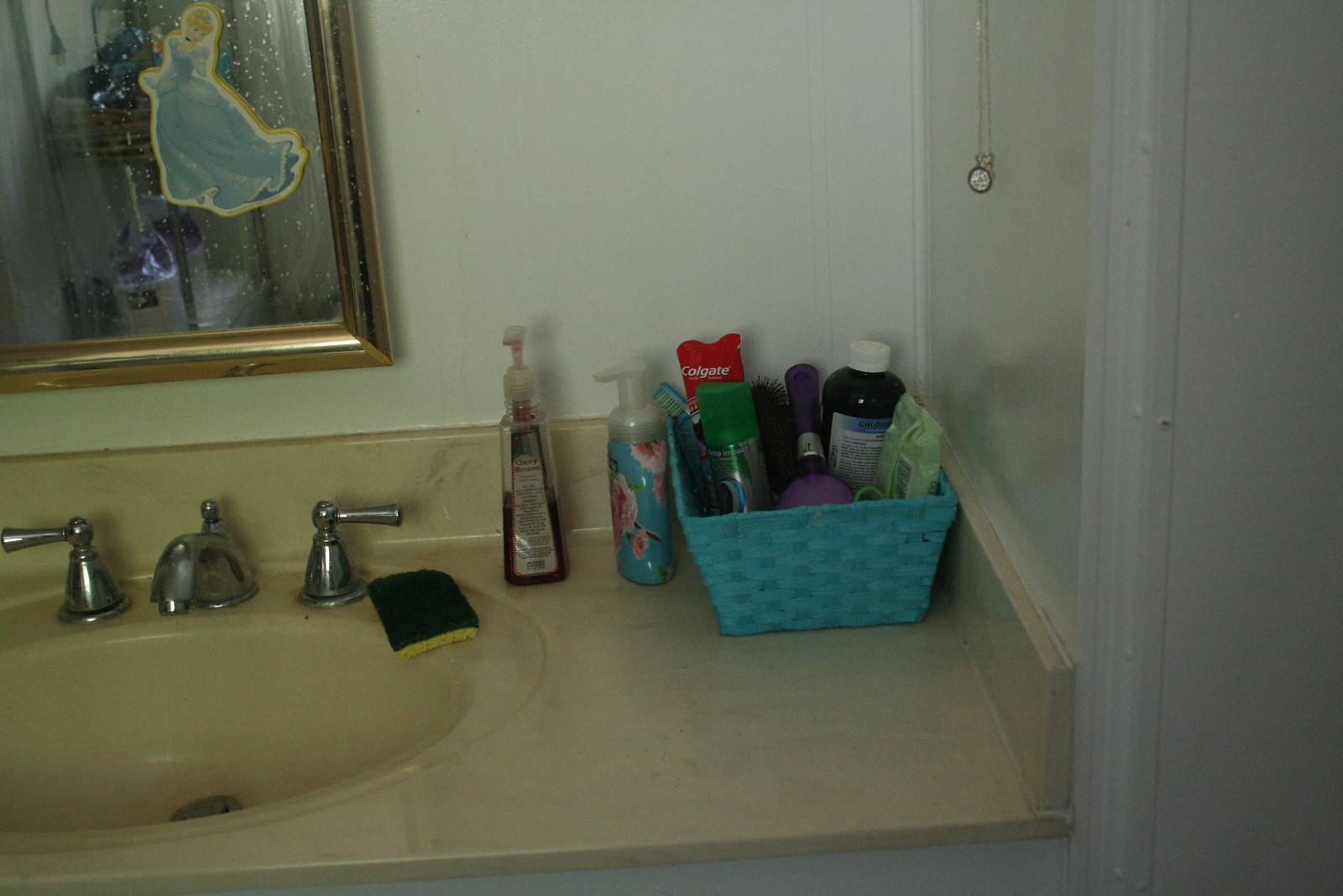The image depicts a well-organized bathroom vanity area featuring a sleek porcelain or marble countertop. Positioned in the corner of the sink is a blue wicker basket, stocked with various bathroom essentials. The countertop houses two hand soaps and a sponge. The sponge has a dark-colored back side and a yellow front side, indicating it is used for scrubbing. The sink itself has two faucet nozzles, designated for hot and cold water. Above the sink, a square mirror is mounted on the wall; however, a section of the mirror appears to be missing, revealing a gray spot. The mirror also reflects an additional item, possibly a shelf, adding to the bathroom’s functional design.